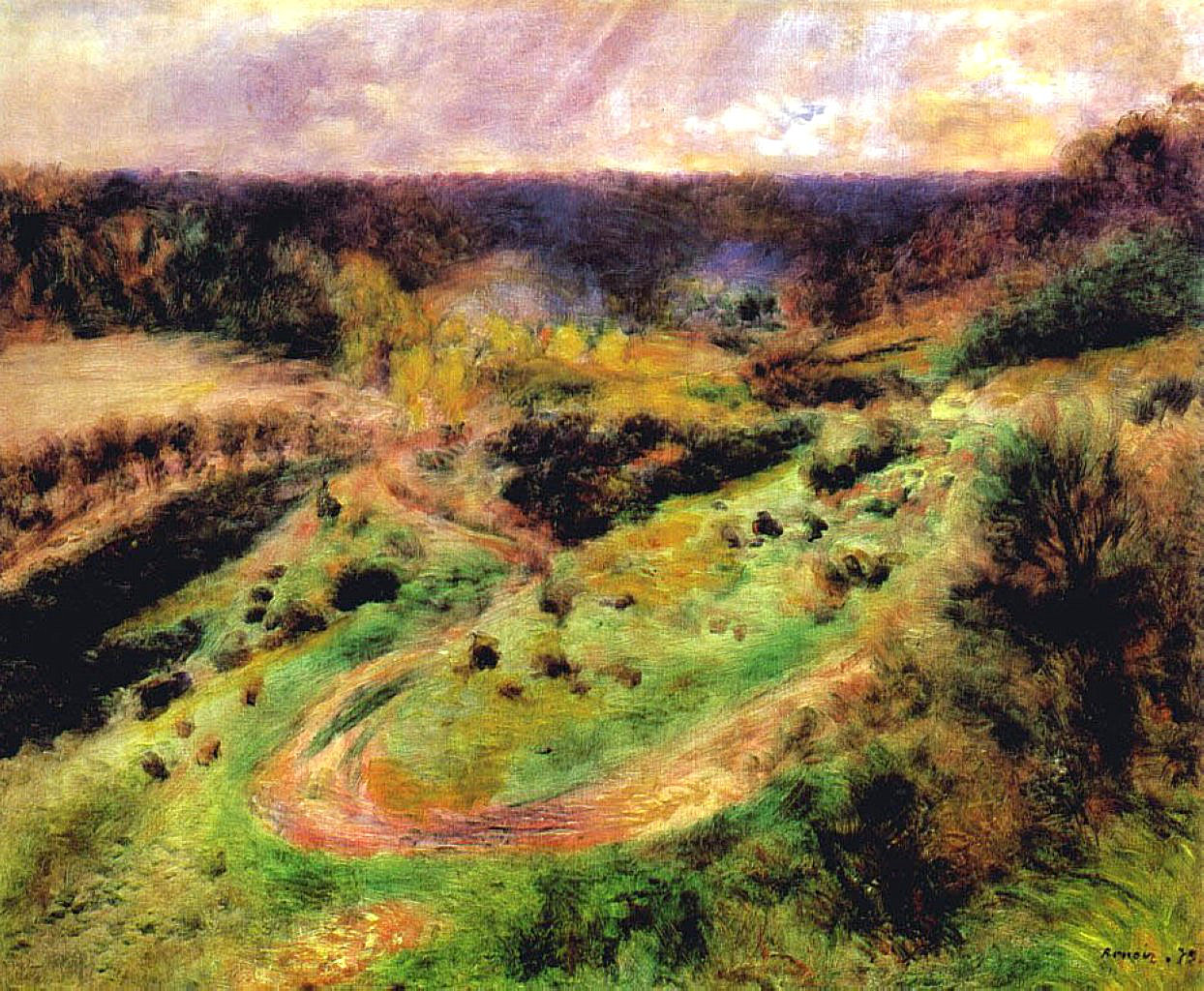This impressionistic painting, signed by the artist in the bottom right corner, showcases a mesmerizing landscape bathed in golden lemon and deep lavender plum hues. The sky is adorned with implied rays of light and sun reflections off the clouds, creating a dreamy ambiance. In the background, the subtle use of purples gives a sense of distant forests and trees, while the foreground warms up with more detailed foliage depicted through heavy brushstrokes and textures reminiscent of chalk or oil pastel.

The scene features a winding dirt road meandering through crested hills adorned with patches of greenery and areas of bush and tree lines. Some trees sport yellow foliage, suggesting an autumn setting. Additionally, the painting includes multi-colored roads and hills, with unique hues of brown, black, and dark green, enhancing its abstract quality. The overall effect is a captivating, somewhat surreal landscape that draws the viewer into its dynamic, colorful world.